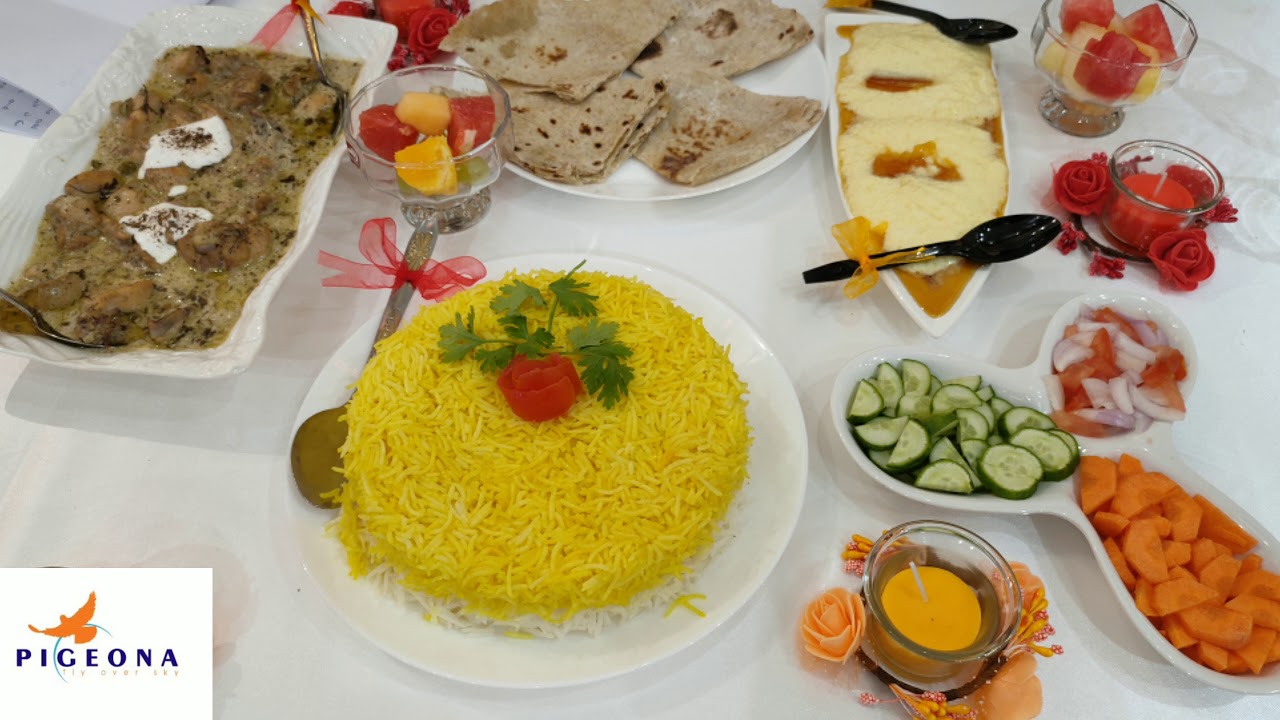This detailed photographic image captures a diverse spread of food items arranged on a white tablecloth, hinting at a well-prepared meal or perhaps a food blogging setup. At the center of the image is a white China plate containing yellow lo mein noodles garnished with a strawberry and parsley sprigs, which is accentuated by a spoon tied with a mesh ribbon. To its right, there is a glass dish featuring an orange flower with an orange candle inside. Above this centerpiece, a white plate is divided into three compartments, showcasing sliced cucumbers, carrots, and onions, arranged in a Y-shaped pattern.

Directly above the lo mein, there is a white plate holding pieces of flatbread, likely chapati or another type of Indian bread. To the right, a dish resembling a white boat holds a pineapple upside-down cake topped with pineapple slices and accompanied by two black spoons adorned with orange ribbons. Nearby is a bowl with red candles and roses, enhancing the visual appeal.

Further to the right, in the top right-hand corner, a glass cup appears to contain pieces of fruit, possibly peaches. To the left of the lo mein, a glass cup filled with strawberries and cantaloupe is situated just above the spoon on the lo mein plate. Adjacent to that, a glass dish presents what looks like a baked goulash dish, brown in color.

In the top left corner, a rectangular white plate or bowl contains a cream and brown curry dish. The bottom left-hand corner of the image features the logo of "Pigeona" with an orange pigeon graphic and the text “Pigeona Fly over sky.”

Together, these elements create a rich and harmonious portrayal of a varied and inviting culinary display, meticulously arranged for an indoor setting.